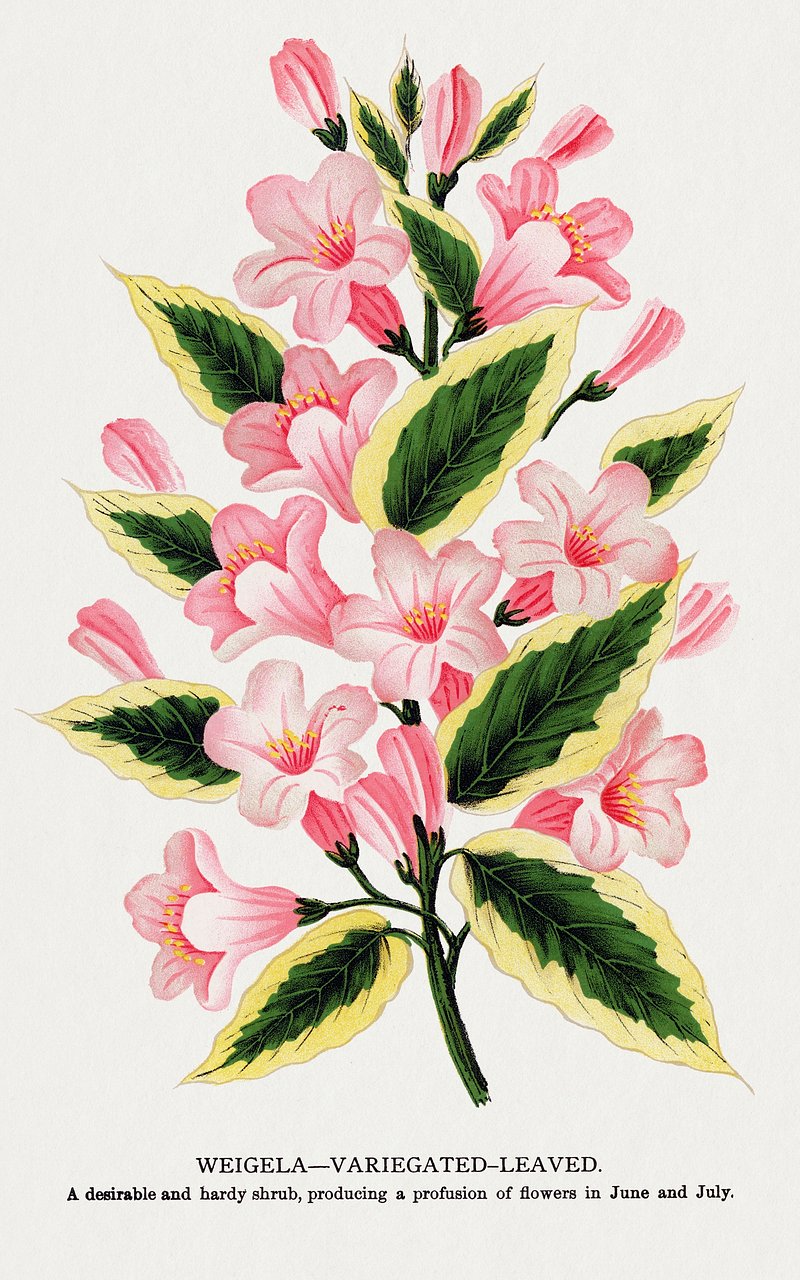The image showcases a detailed hand-drawn or possibly watercolor artistic print of a beautiful flowering shrub known as Weigela variegated leaved. The illustration is featured on an off-white to light gray rectangular paper background without a border. At the bottom of the piece, there is a descriptive black text that reads: "Weigela variegated leaved, a desirable and hardy shrub producing a profusion of flowers in June and July."

The central focus of the image is the shrub's stem, which supports multiple green leaves with a light yellow or creamy tan border. Around ten trumpet-shaped pink flowers adorn the stem, each exhibiting a darker base transitioning into lighter petals. The intricate depiction captures the delicate nature of the flowers and the variegation of the leaves, emphasizing the plant's lush and vibrant appearance, reminiscent of a gladiola's growth pattern.